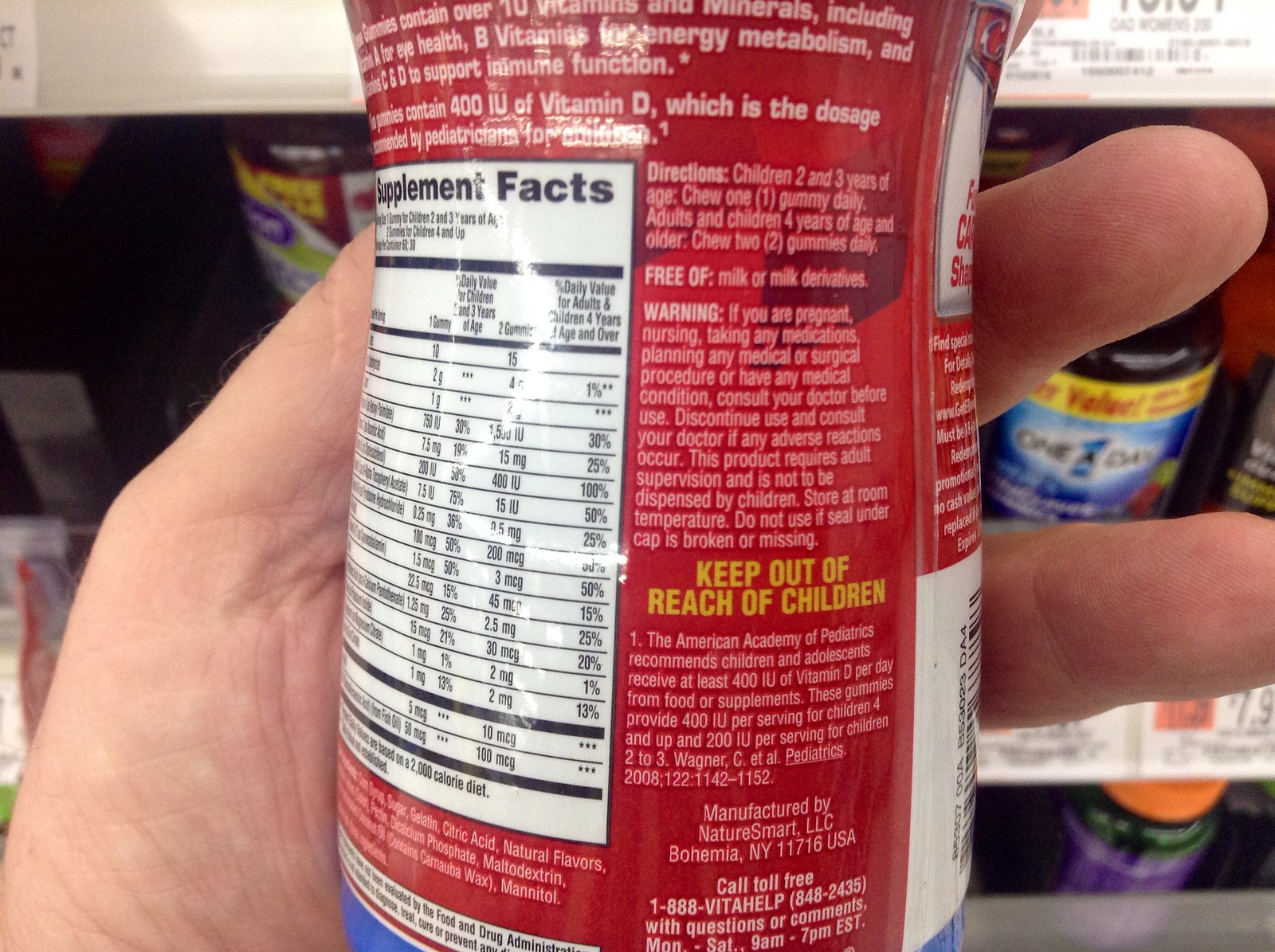A person is holding up a red bottle with a detailed label in a store aisle that appears to be the vitamins and supplements section. The label features a variety of information, including nutritional facts displayed on a white block with black lettering on the left side of the bottle. At the top of the label, there is more information about the contents of the bottle. Directions on the red section advise that children aged 2 to 3 should chew one gummy daily, whereas adults and children 4 years and older should chew two gummies a day. The label also states that the product is free of milk and milk derivatives, and includes a caution in yellow text to keep the product out of reach of children. Below this warning, the label details the manufacturing information: "Nature Smart LLC, Bohemia, New York, 11716 USA," along with a toll-free number for VitaHelp (1-888-VITA-HELP). The background of the image shows a blue one-a-day vitamin bottle, along with beige shelving strips equipped with white price tags edged in salmon color, enhancing the context of being in a vitamin aisle.